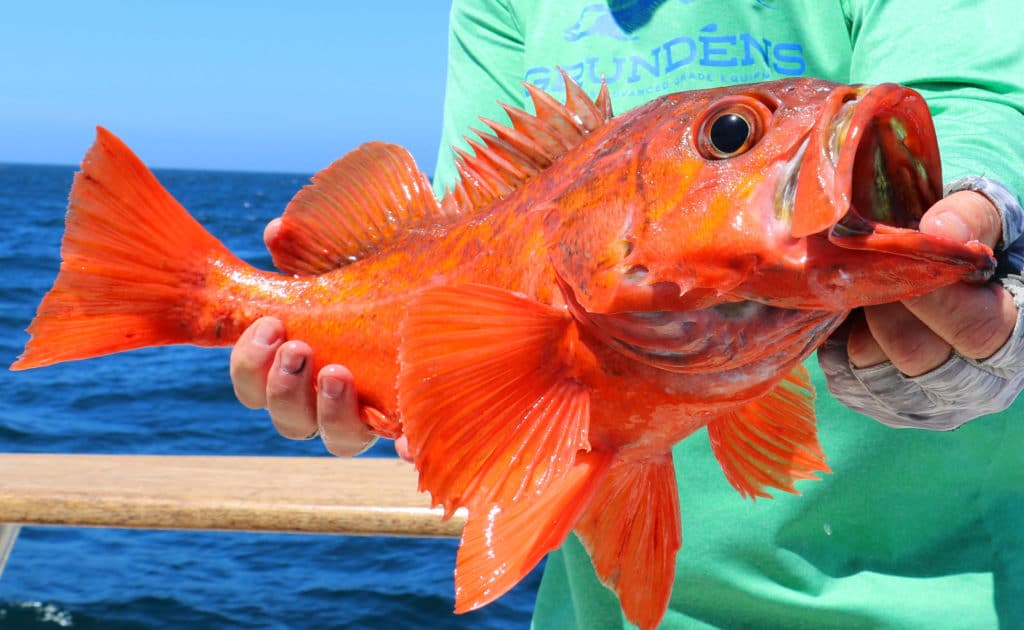This photograph captures a person standing by the railing of a boat, against a backdrop of turquoise blue ocean water under a light blue sky with visible waves. The scene is set outdoors, possibly on a fishing trip. We can only see the individual from the neck down to the waist, clad in a light green long sleeve shirt or apron that bears the blue lettering "Grundon's" on the chest. The person, who appears to be a Caucasian male, is wearing fingerless gloves on his left hand, which is gripping a large, vibrant orange fish. The fish, resembling a goldfish with medium dark orange coloring, has distinct fins and a spiky dorsal fin, round black eyes, and an open mouth that is being held by the person. The fish's vivid orange contrasts sharply with the bright, clear blue of the ocean water in the background, creating a striking visual image.